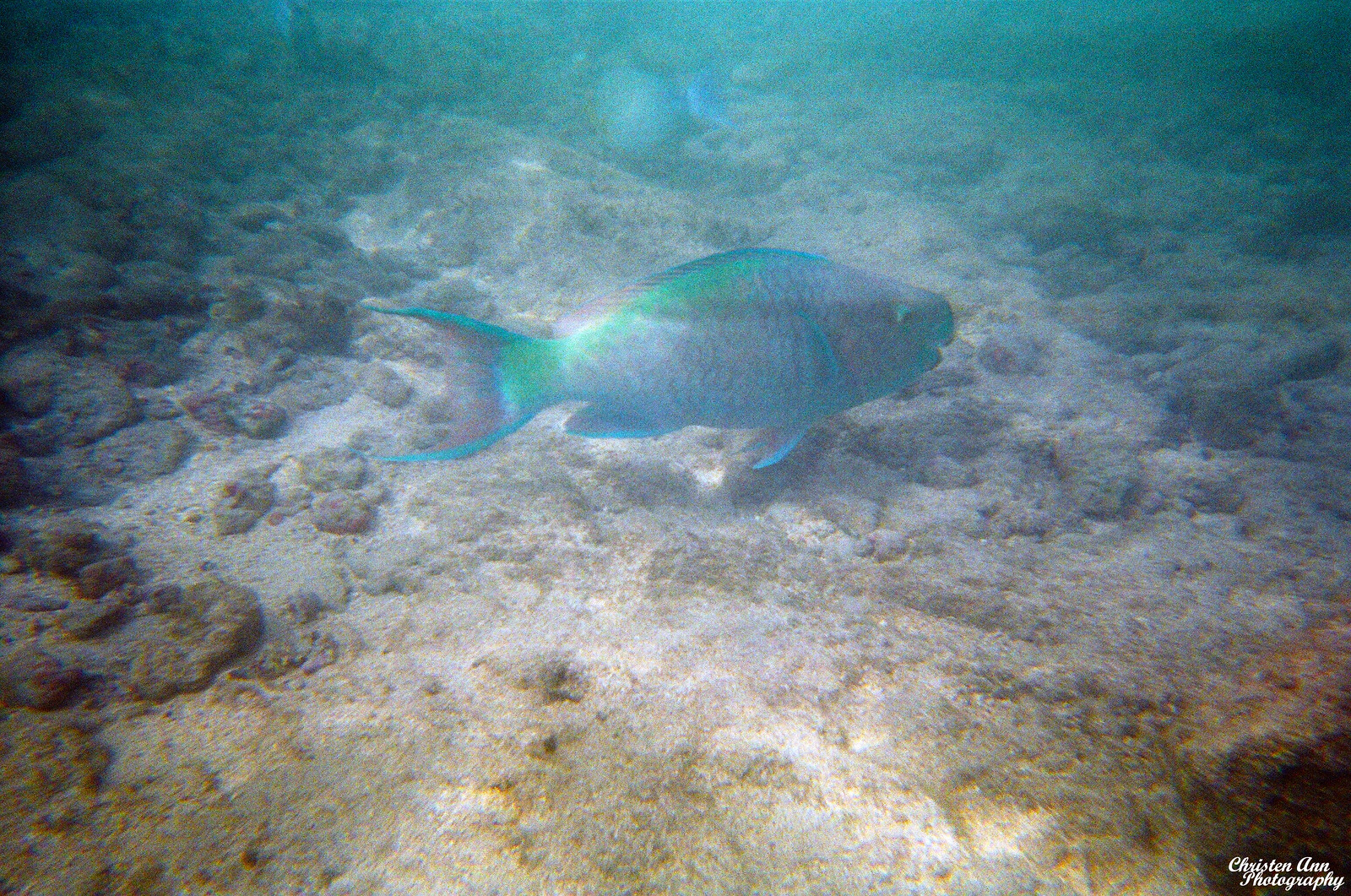This underwater photograph, approximately four inches tall and six inches wide, features a striking blue fish prominently positioned near the center. The fish, possibly a parrotfish, showcases an array of mesmerizing colors: a vivid blue mouth and fins, a blue and black dorsal fin, and an emerald green band along its side that extends to its tail, which fanned out into two long, blue-tipped points. Intriguingly, a thin band of brownish-pink punctuates the tail. The fish's body also exhibits scales with shades of purple, gray, and possibly brown.

The setting appears to be either the ocean floor or an aquarium, with the sandy ground below the fish displaying hues of light brown and gray, interspersed with rocks and sediment. A darker patch marks the lower right corner of the image. The rock bed beneath the fish shows a progression from a dark greenish tint to a lighter gray, transitioning to an almost greenish-white and gray in the forefront. The photograph is marked by "Kristen Anne Photography" in white cursive at the lower left corner.

The background features a faded greenish-blue ambiance, hinting at the underwater environment. There may be additional, albeit blurry, fish visible in the distance. A light source softly illuminates the upper back of the fish and the corresponding area on the rocky bed, adding to the surreal, almost magical quality of the underwater scene. The fish seems intent and purposeful, as if it might be swimming towards us, possibly in search of food.